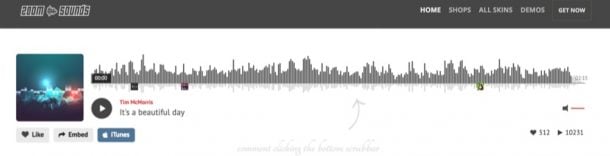This image displays a screenshot of a website called Zoom Sounds, a platform geared towards musicians and music enthusiasts. The Home category is selected from the right-hand side menu, which also includes options like Shops, All Skins, Demos, and Get Now. Central to the page is a song being played, entitled "It's a Beautiful Day." Although the name of the artist, written in small orange text above the title, is somewhat difficult to discern, it appears to be either Tim McMorris or Tim McHarris. The accompanying image for the song is a dark blue nighttime sky adorned with clouds in vibrant neon red and blue hues. A striking feature is a neon blue cloud that seems to emit a shooting star or light. Additional features on the page include buttons to like, embed, or purchase the track on iTunes. The song has garnered significant attention, with 512 likes and 10,231 listens.